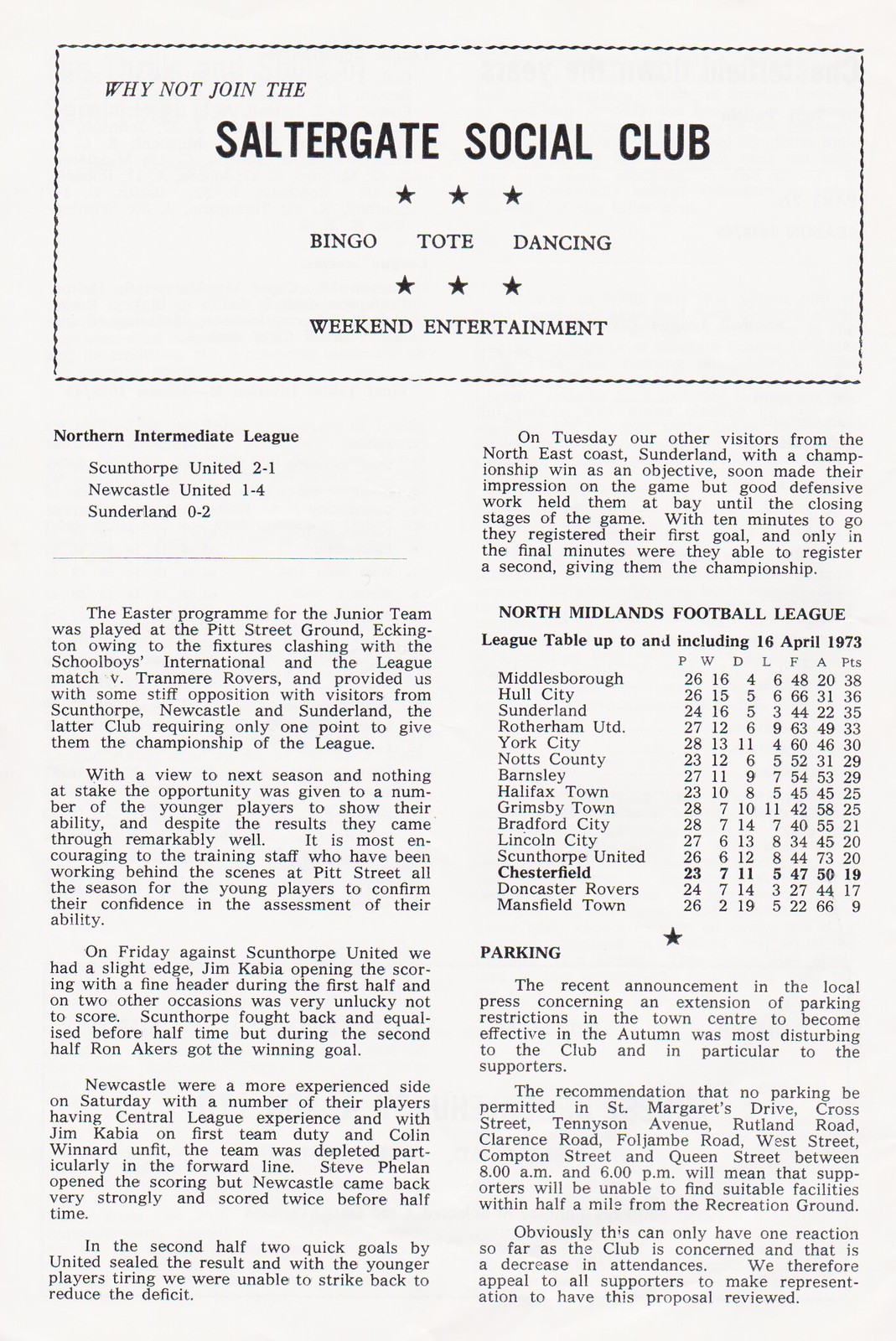This image displays a screenshot of a page from what appears to be a book, magazine, or brochure. The page features a clean white background with a thin black-framed rectangle at the top. The black text within this rectangle reads, "Why Not Join the Saltergate Social Club?". Below this title, three five-pointed black stars are followed by the words, "bingo, tote, dancing". Another trio of black stars follows before it continues with "weekend entertainment".

The main body of the page is divided into two columns. The left column starts with an infograph chart titled "Northern Intermediate League", listing scores such as Scunthorpe United 2-1, Newcastle United 1-4, and Sunderland 0-2. Underneath this chart, an article occupies the rest of the column, running down to the bottom of the page.

In the right column, a paragraph of text is followed by another highlighted section in bold letters: "North Midlands Football League, league table up to and including 16 April, 1973". This section continues to present details of the leagues and a series of scores, providing a comprehensive overview of football standings up to the specified date.